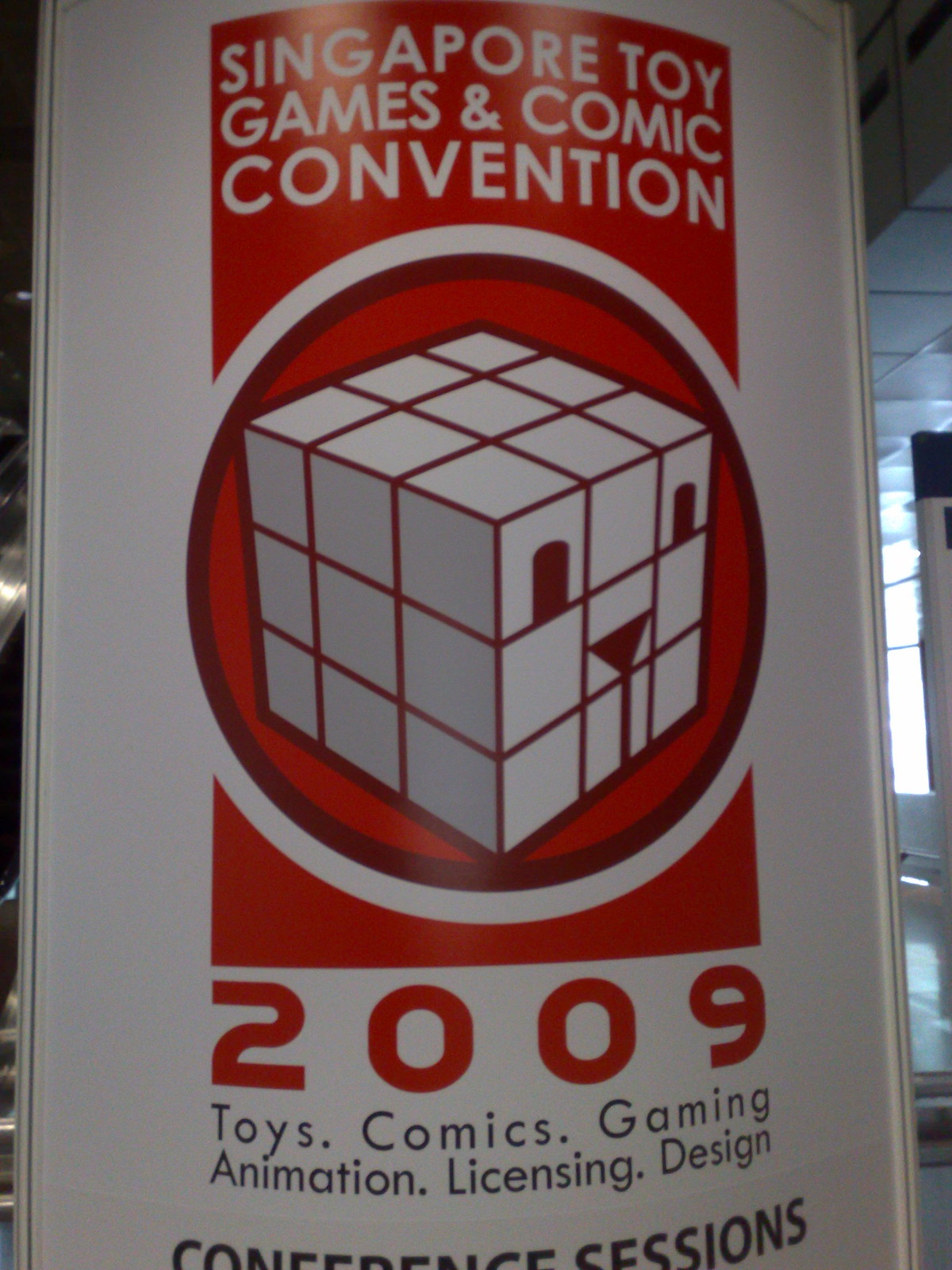The image depicts an indoor banner, likely mounted on a wall or pole, promoting the Singapore Toy, Games, and Comic Convention 2009. Dominating the center is a red vertical rectangle with a white circle intersecting it. Inside the circle, a 3x3x3 white cube, resembling a Rubik's Cube, features a face with eyes and a nose on its right face. At the top of the rectangle, in prominent white lettering, the text reads "Singapore Toy, Games and Comic Convention." Beneath that, in red font, is the year "2009," followed by a list of event highlights in black text: "Toys, Comics, Gaming, Animation, Licensing, Design." The final line mentions "Conference Sessions" and is also in black. The overall setting is indoors with visible windows and walkways, and the lighting is notably low.